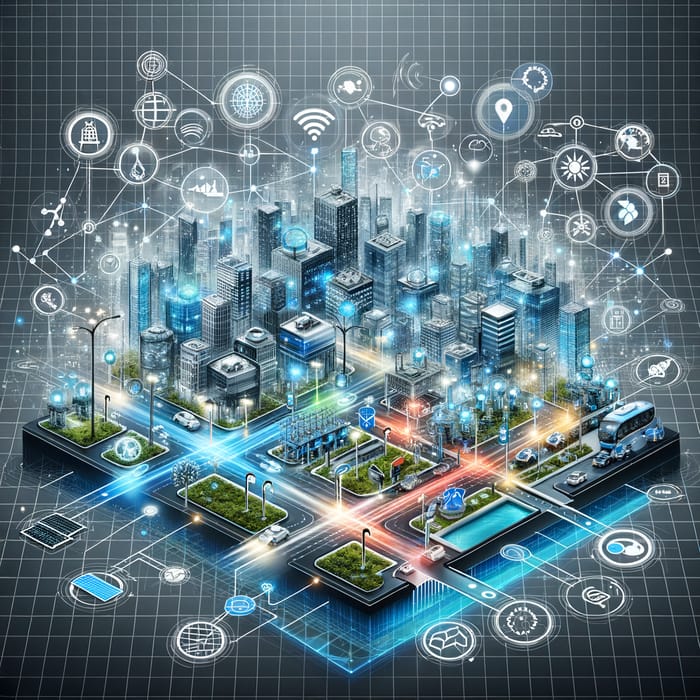The image is a detailed computer-generated illustration of a futuristic city presented in a vertical, rectangular shape. The cityscape is composed of tall high-rise buildings, roads, and green spaces, all depicted on a gray and white grid pattern that serves as the background. The entire city is enveloped in a network of interconnected, circular icons, each representing different aspects of connectivity such as Wi-Fi, internet activity, or miscellaneous digital symbols. These icons are uniformly arranged in blue, yellow, and orange, with white lines linking them to represent the web of connections. Additionally, the graphic includes various labels denoting specific elements like cars, traffic lights, and areas with Wi-Fi access, all enhancing the intricate and interconnected nature of this urban landscape. The overall effect is a highly detailed and visually engaging portrayal of a smart city integrated with digital networks and modern amenities.